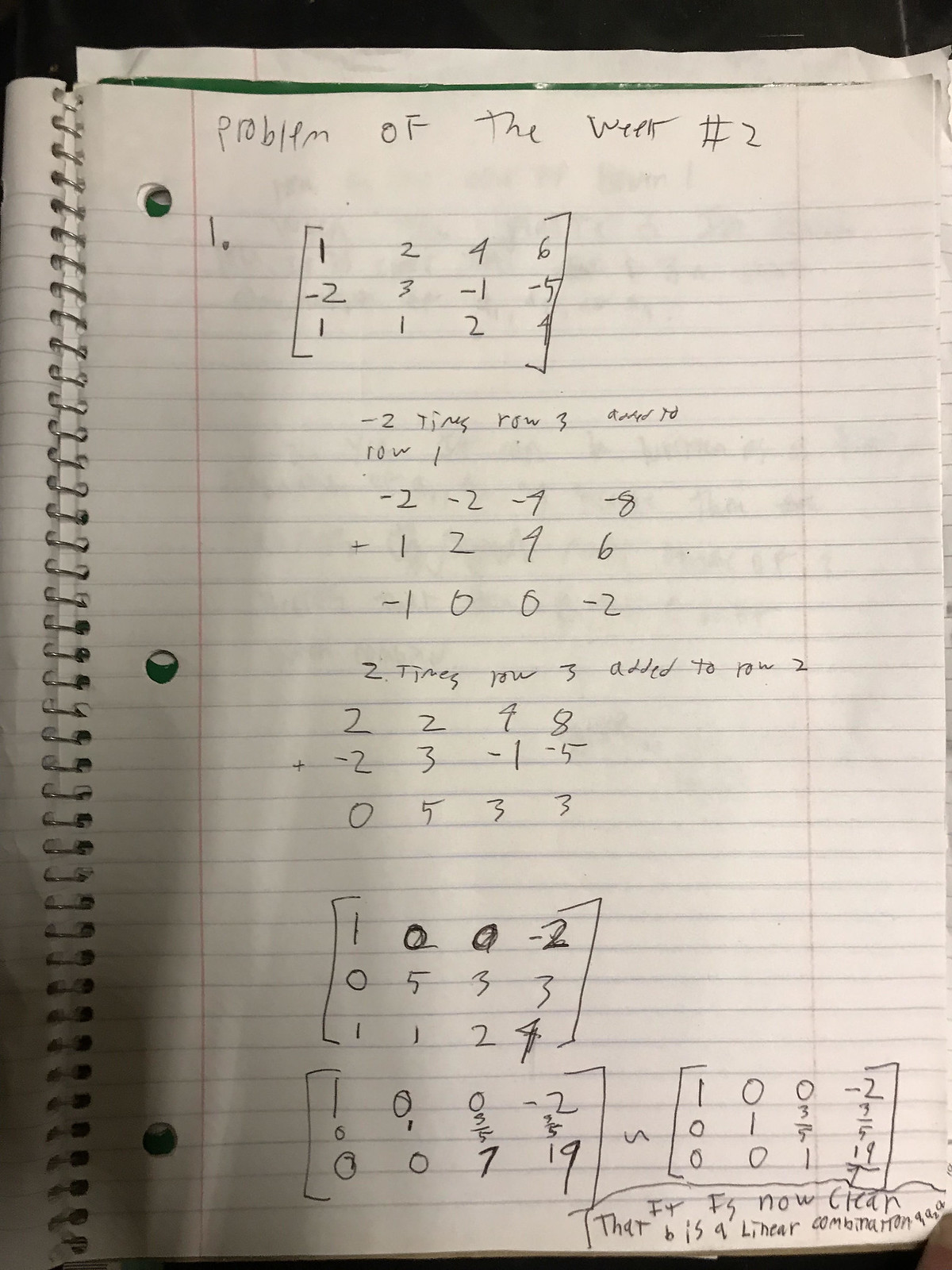The image features a vivid green spiral-bound notebook placed against a stark black background. The notebook is opened to a page with white paper that has blue horizontal lines and red vertical margins on both sides. At the top of the page, in prominent handwriting, it reads "Problem of the Week," followed by "Number 2." Below this heading, the notebook is filled with various rows of numbers and mathematical notations arranged sequentially.

The first line starts with "1" followed by "1, 2, 4, 6." On the next line, a sequence of numbers includes "-2, 3, -1, -5," followed by another set of figures, "1, 1, 2, 4." Continuing, additional mathematical expressions are written, including "-2 times row 3," and sequences like "-2, -2, -4, -8," and "1, 2, 4, 6." Further down, there appears to be a line of results, "-1, 0, 0, -2."

The detailed linear notations and sequences of numbers continue to fill the page, indicating a complex mathematical problem. On the bottom of the page, there is a small, barely legible note with unclear handwriting. It appears to reference some additional linear equations or instructions, but the poor legibility makes it difficult to decipher.